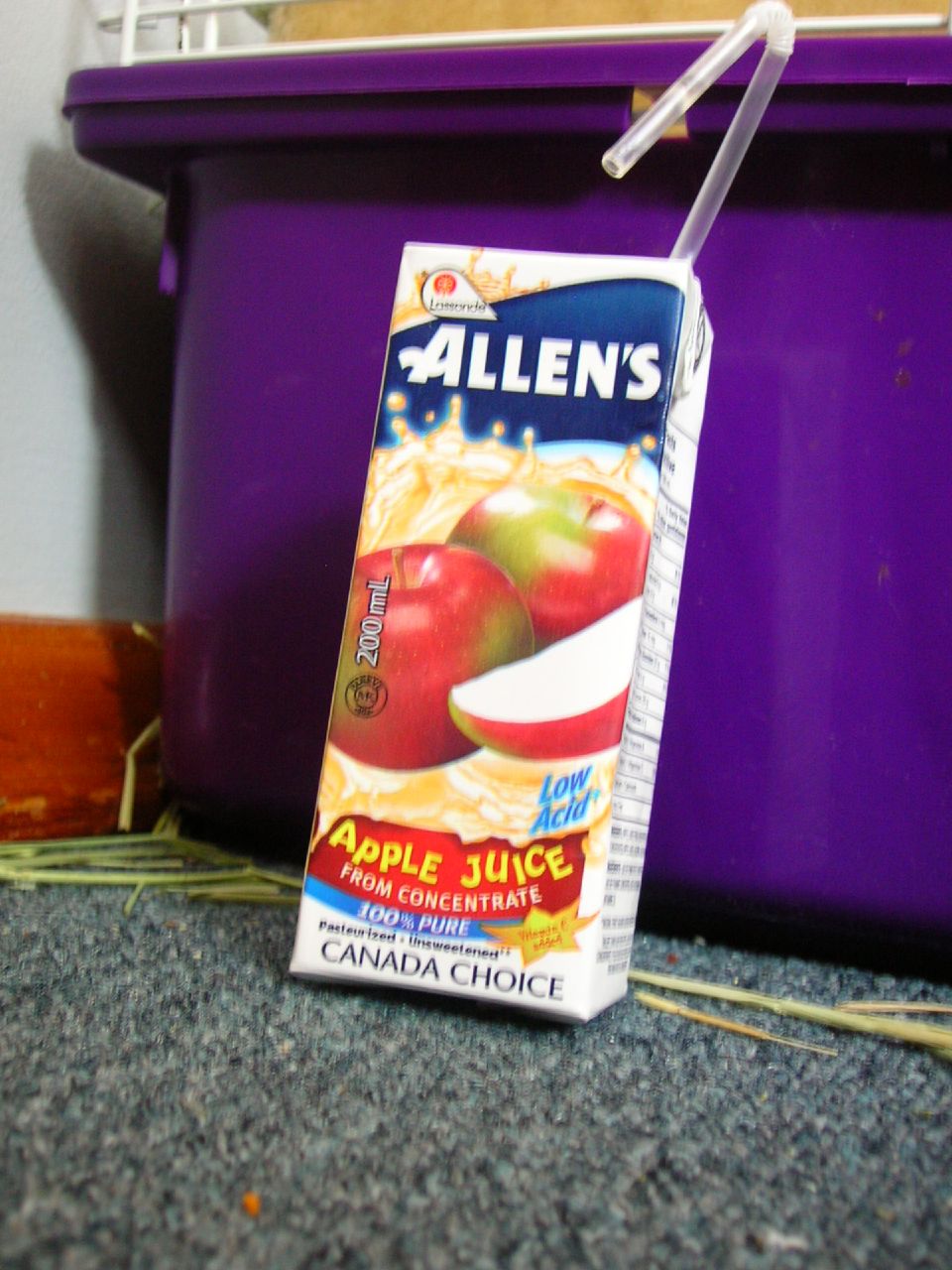The image captures a prominently featured Allen's Apple Juice box, which is white with blue and gold accents and adorned with illustrations of green and red apples. The box clearly states "Apple Juice from Concentrate," "100% pure," and "Canada choice," with additional mentions of it being low acid, pasteurized, and unsweetened. A clear straw is inserted into the top of the juice box, indicating it has been opened.

The juice box is leaning at an angle against a bright purple plastic tub. This tub has a white cage placed on top and is situated in front of a wooden structure in the background. The scene is set against a white wall with a brownish-red three-inch baseboard along the bottom. The floor is covered with a bluish-gray Berber carpet that has scattered strands of dried hay or wheat.

The lighting in the image is bright, emphasizing the juice box as the main focal point, and casting noticeable shadows onto the purple tub behind it. The meticulous details of the juice box's text, the colors, and the surrounding environment are clearly visible, making the composition both vivid and informative.